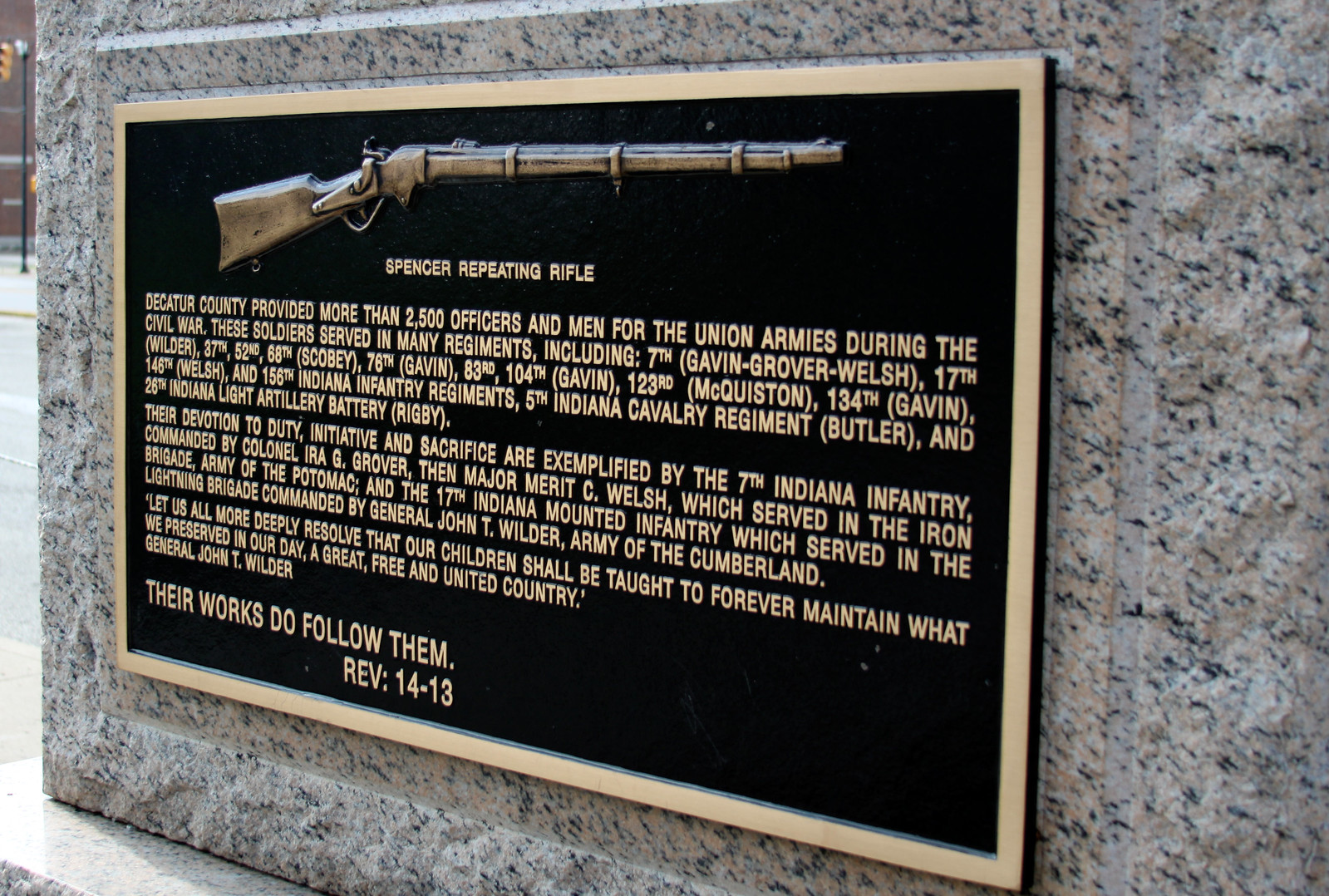The image depicts a commemorative plaque mounted on a piece of whitish-gray flecked granite with dark lines running through it, resembling a monument. The plaque has a black background with gold or bronze lettering and is bordered by a gold edge. At the top of the plaque is a bronze or brass relief of a Spencer Repeating Rifle. Below the rifle, the plaque provides an inscription explaining the historical significance of this firearm, detailing how it was used by officers and men of the Union armies during the Civil War, particularly mentioning Decatur County, which provided over 250 soldiers. These soldiers served in various regiments, and the text elaborates on their contributions. At the bottom of the plaque, in larger gold letters, is the quote "Their works do follow them, Rev. 14-13." The plaque appears to be part of an outdoor monument, potentially located in a cityscape with a thin stoplight visible in the background.